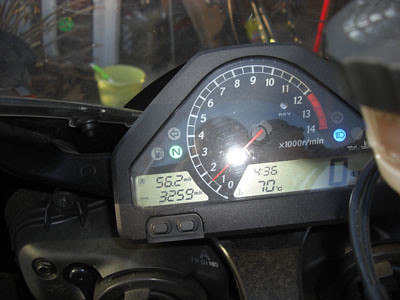This photograph captures a detailed view of a speedometer on a mechanical device, likely a vehicle dashboard, within a garage setting. The large, circular speedometer dial ranges from 0 to 14, with a red danger zone marked between 12 and 14. The current speed is indicated by a red arrow, which points to 1.5 thousand revolutions per minute (rpm). 

Beneath the speedometer dial, there is a digital clock displaying the time as 4:36, and a temperature reading of 70 degrees. To the left of the speedometer, another digital window shows readings of 56.2 and 32.59, possibly indicating accumulated mileage or other metrics. An illuminated "N" can be seen on the dashboard, which could suggest the vehicle is in neutral. Additional indicators include a small fuel gauge and turn signal arrows.

The background reveals the vehicle is parked in a garage, evidenced by the visible window through which a glass cabinet filled with various items can be seen. A yellow bucket and miscellaneous objects are scattered on the garage floor, reinforcing that the vehicle is stationary but still has its instrument panel lit up.